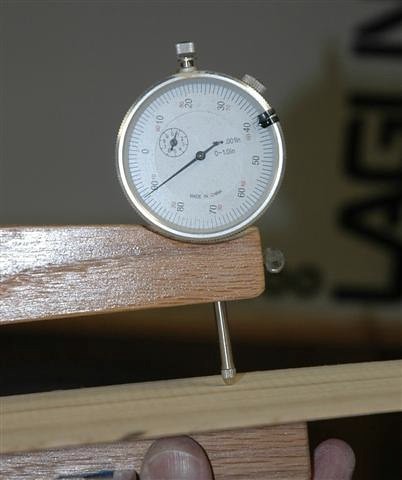A detailed close-up image of a small, round timepiece, possibly a stopwatch, featuring a silver rim and a button on the right side that protrudes significantly—a common feature of stopwatches. Next to this button is a small knob likely used for calibration. To the right of the knob, two black clips are attached to the stopwatch's rim. The timepiece appears to be mounted or resting on a wooden surface that resembles the leg of a chair. Extending from the bottom of the wooden support is a long metal stem, which could either be part of the stopwatch or an external attachment, adding an element of ambiguity to the device's exact nature.